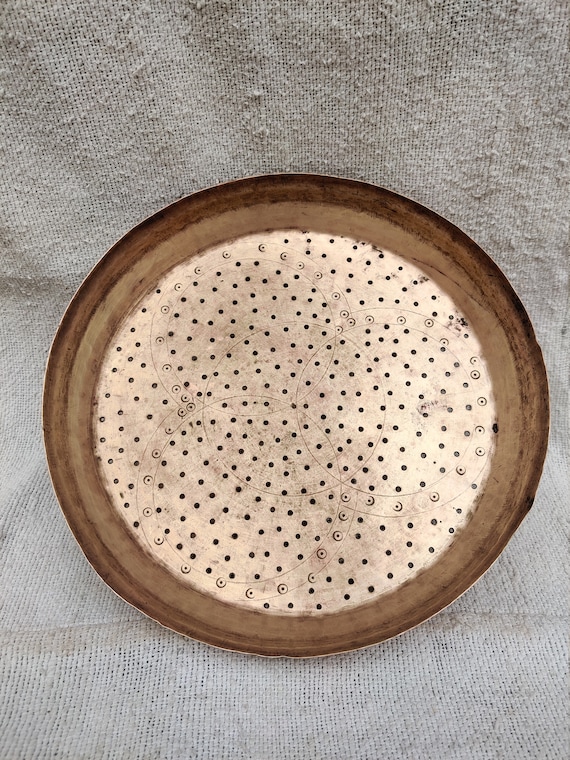The image displays a unique, circular object prominently set against a light gray canvas-like fabric background. The object features a dark brown wooden rim encircling a metal center, which is adorned with a spirograph-like geometric pattern. This pattern consists of multiple medium-sized circles interconnected, etched into the off-white metal surface. The entire metal area is punctuated by evenly spaced pinholes, suggesting potential uses like a pin cushion or some astronomical or astrological tool. The intricate design and uniform pinholes, along with the craftsmanship in metal and wood, imply it could also be a custom-made serving tray. The detailed combination of wood and etched metal gives it an unusual yet intriguing appearance not commonly seen.